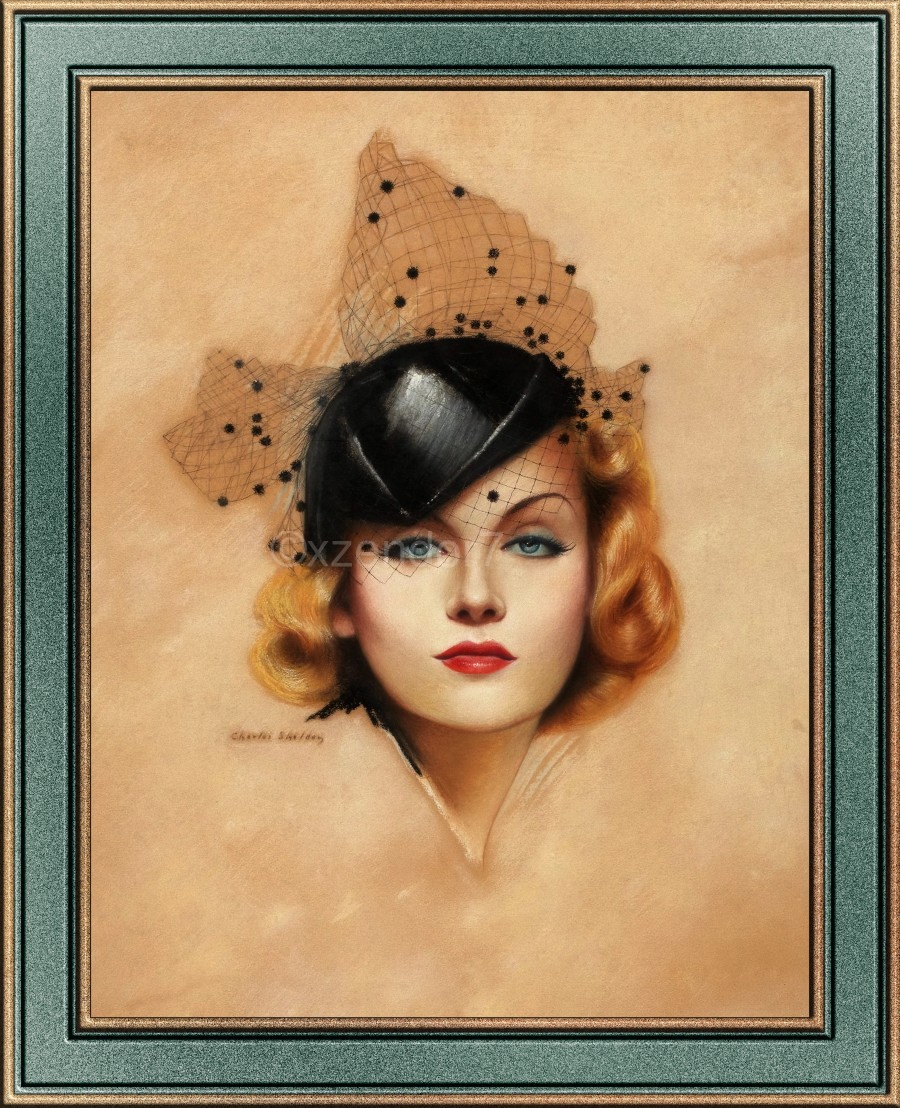The image is a framed, portrait-oriented painting with a dark aqua wooden frame edged with gold. Within the painting, the background exhibits a mottled creamy beige pattern. Centrally positioned, the subject is the face and neck of a woman with light skin, adorned with heavy eye makeup and vibrant red lipstick. She has chin-length, wavy blondish-red hair, styled in a 40s or 50s fashion. Her arched eyebrows match her well-defined features. The woman wears a tilted black hat, likely a pillbox style, adorned with a black mesh net featuring black dots typical of the period, covering part of her face. A significant detail also includes a large, light brown bow with black spots, positioned at the back of the hat. She gazes directly at the viewer with piercing bluish-green eyes, giving the painting a captivating focus. Near the bottom left of her facial area, the artist's signature is visible.